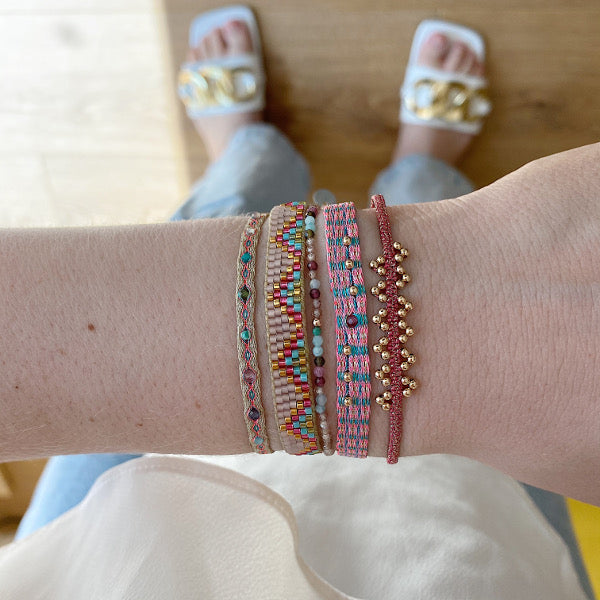The image captures a close-up of a light-skinned woman's left wrist adorned with five distinct handmade bracelets. Each bracelet showcases a unique design and texture, contributing to a colorful and eclectic ensemble. One bracelet features a dainty strand of beads, while another stands out with a red band embellished with spherical gold beads. There is also a bracelet with threads of pink, blue, and white, interwoven with beads, and two other woven bracelets include mixes of tan, turquoise, and red elements. The woman's wrist, displaying a few freckles, is set against the backdrop of her outfit—a white blouse, light blue denim capris, and white slide-on sandals with gold circle accents. The photograph, seemingly taken indoors, focuses primarily on the vibrant and diverse bracelets, with the rest of her attire and surroundings slightly blurred.